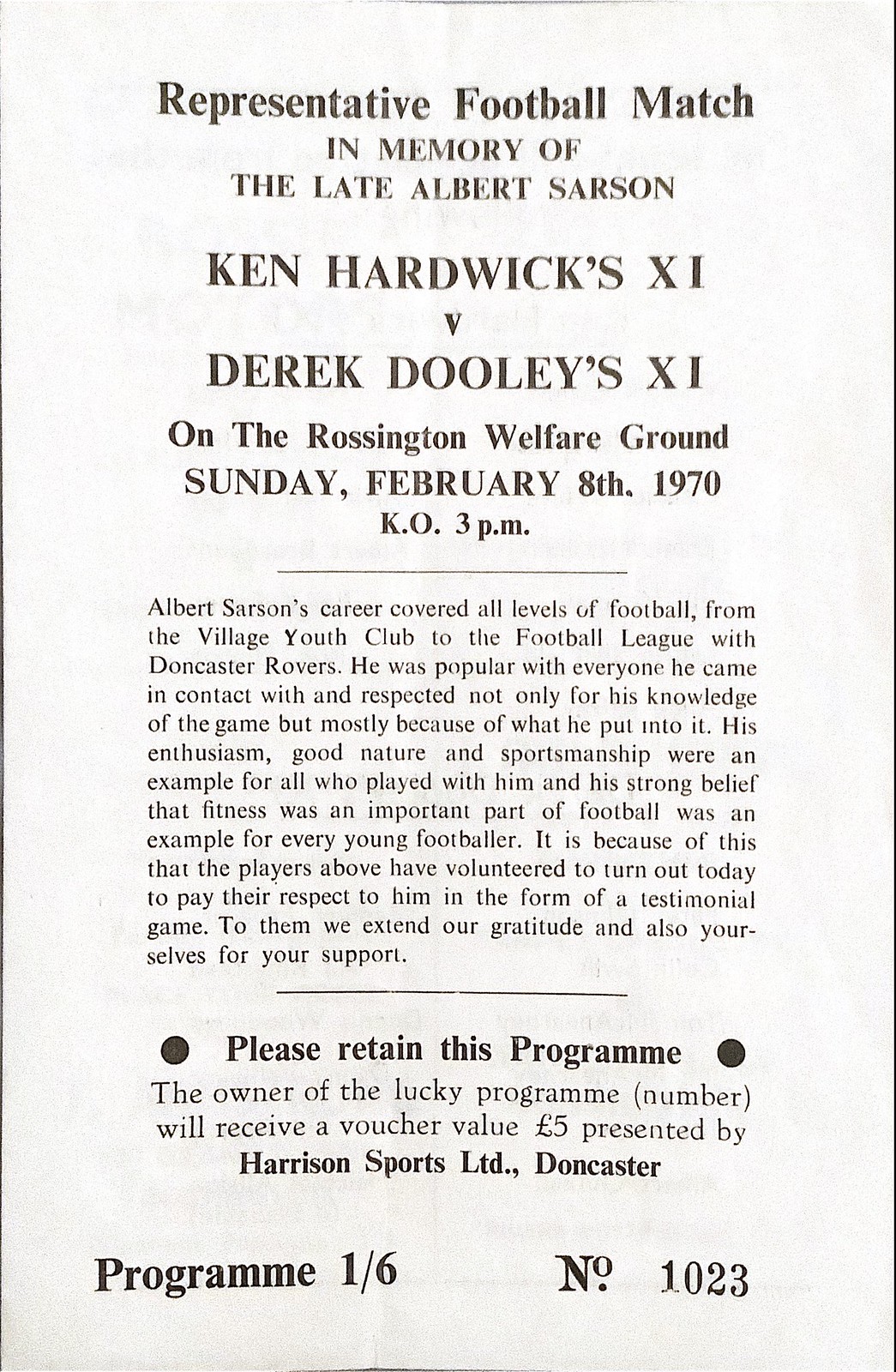This black and white image appears to be a snippet from a magazine or a presentation sheet, featuring a white background with typed black text. There is a thin border on the left and right sides. The text at the top announces a "Representative Football Match in Memory of the Late Albert Sarsen," with Ken Hardwick's XI facing Derek Dooley's XI. The match is scheduled to take place at the Rossington Welfare Ground on Sunday, February 8, 1970, with a kickoff at 3 p.m. 

The middle section, though hard to read, provides background information on Albert Sarsen's career, noting his contributions to various levels of football, including the Football League with Doncaster Rovers. He was admired for his knowledge of the game, enthusiasm, good nature, sportsmanship, and advocacy for fitness. The match is described as a testimonial game held in his honor.

At the bottom of the page, there is a note instructing attendees to retain their program, as the owner of the lucky program number 1023 will receive a voucher valued at five pounds, presented by Harrison Sports Ltd. of Doncaster. The program is marked as "1-6 number 1023."